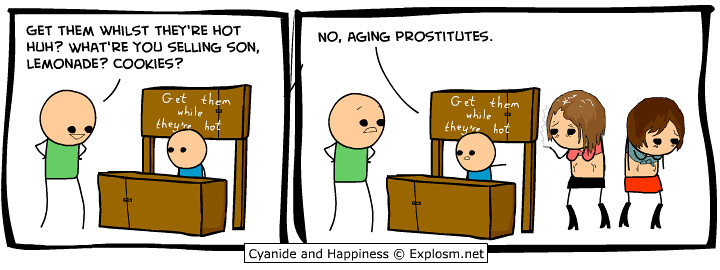The comic features two panels with a white background framed in black. In the first panel, a character with a peach-colored round head, dark circles for eyes, an upside-down triangle for a mouth, a rectangular green torso, and stick arms and legs stands in front of a brown cardboard lemonade stand with a sign that reads "Get them while they're hot" in white lettering. This character is speaking, saying, "Get them whilst they're hot, huh? What are you selling, son? Lemonade? Cookies?" The stand is occupied by another character with a peach-colored head, dark circles for eyes, and a blue torso.

In the second panel, the same green-torsoed character points towards two older-looking women on the right. These women have lined faces and bodies, indicating age, and are wearing tank bikini tops (one red, one blue) with sagging breasts, black skirts, and black knee-high boots. The text at the top of this frame reads, "No, aging prostitutes." The comic is captioned at the bottom in a white rectangle with black lettering: "Cyanide and Happiness © explosm.net."